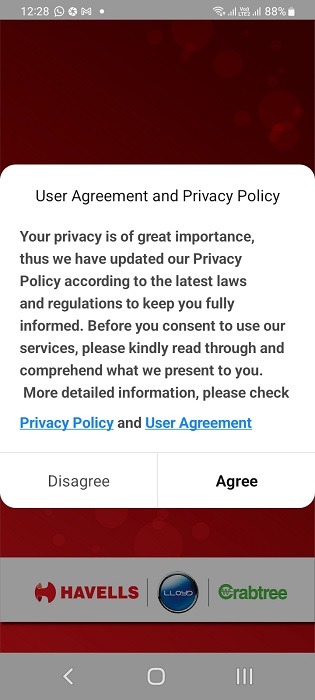The image displays a screenshot of a website on a mobile device, characterized by a thin gray status bar at the top. The status bar includes several icons: the time "12:28," followed by a phone symbol, a cogwheel, an "M," and a dot. To the right side of the banner, signal indicators show the cell signal strength, Wi-Fi strength, "LTE 2," and a battery icon indicating 88% charge.

The main section of the image has a burgundy red background, overlaid by a pop-up notification in a gradient of gray to white. The notification text, in a light black to charcoal gray font, reads: "User Agreement Privacy Policy. Your privacy is of great importance. Thus, we have updated our privacy policy according to the latest laws and regulations to keep you fully informed. Before you consent to use our services, please kindly read through and comprehend what we present to you. For detailed information, please check Privacy Policy and User Agreement." The phrases "Privacy Policy" and "User Agreement" are hyperlinked in blue text.

Below the text, on the left, there is a "Disagree" button, while on the right, there is an "Agree" button in bold black text. In the background, partially visible through the pop-up, is the text "HAVLs" set inside a blue circle with additional lettering. Further to the right, the word "Crabtree" appears in green print with a capital "C."